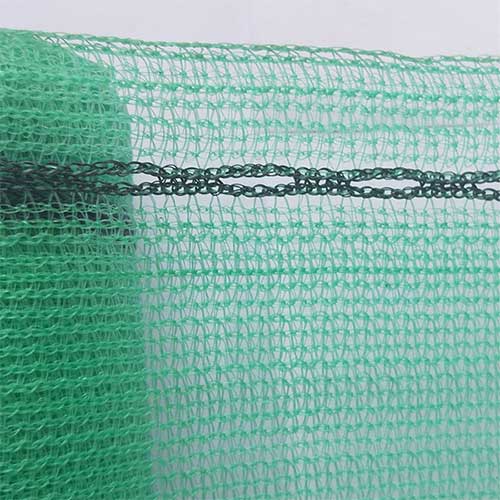This close-up image features a green mesh textile displayed in front of a light gray background. On the left side of the image, the fabric is tightly bundled and appears more opaque against what might be a solid white background. The right two-thirds of the image showcase the mesh textile more distinctly, with the light gray background visible through its woven structure. The mesh is considerably thin, akin to a type of plastic wrap, often found in home improvement stores. A distinct black seam runs across the upper third of the image, likely serving as the hem double-stitch reinforcement along the edge. The entire object captured occupies almost the entire frame, highlighting its woven, grid-like pattern interspersed with shades of green and accentuated by the black seam.